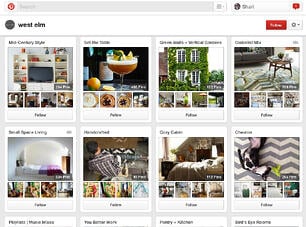The image depicts a Pinterest user interface. On the left side, there is the Pinterest logo, a white 'P' inside a red circle, followed by a prominent search bar. To the right, there's a small circle with a profile image, although it's dark and hard to discern. The screen name beside it reads "SHARI," accompanied by a red notification square with the number '1'. 

Below the header, in lowercase black text, it says “west elm,” with an option to follow displayed in a red square to the right. The Pinterest board showcases various categorized pins, prominently featuring the following:

1. **Mid-Century Style:** An image displaying a television set within a bookcase that is adorned with numerous decorations, including orange and yellow vases and plants.
   
2. **Set the Table:** This category displays an inviting image of a mixed drink garnished with lemon slices, set against a background with green walls and vertical gardens.

3. **Globalist Mix:** This section is to the right of the aforementioned categories.

4. **Small Space Living:** Located at the bottom left, showcasing creative ideas for compact living areas.

5. **Handcrafted:** Featuring artisan craftsmanship and DIY projects.

6. **Cozy Cabin:** Displays a warm, inviting scene with a fireplace, blanket, and couch, perfect for a snug cabin atmosphere.

7. **Chevron:** Features a white and gray zigzag print rug with a dog lounging on it. This category has 265 pins.

Each section is represented with vivid imagery, reflecting a variety of lifestyle and home decor inspirations.